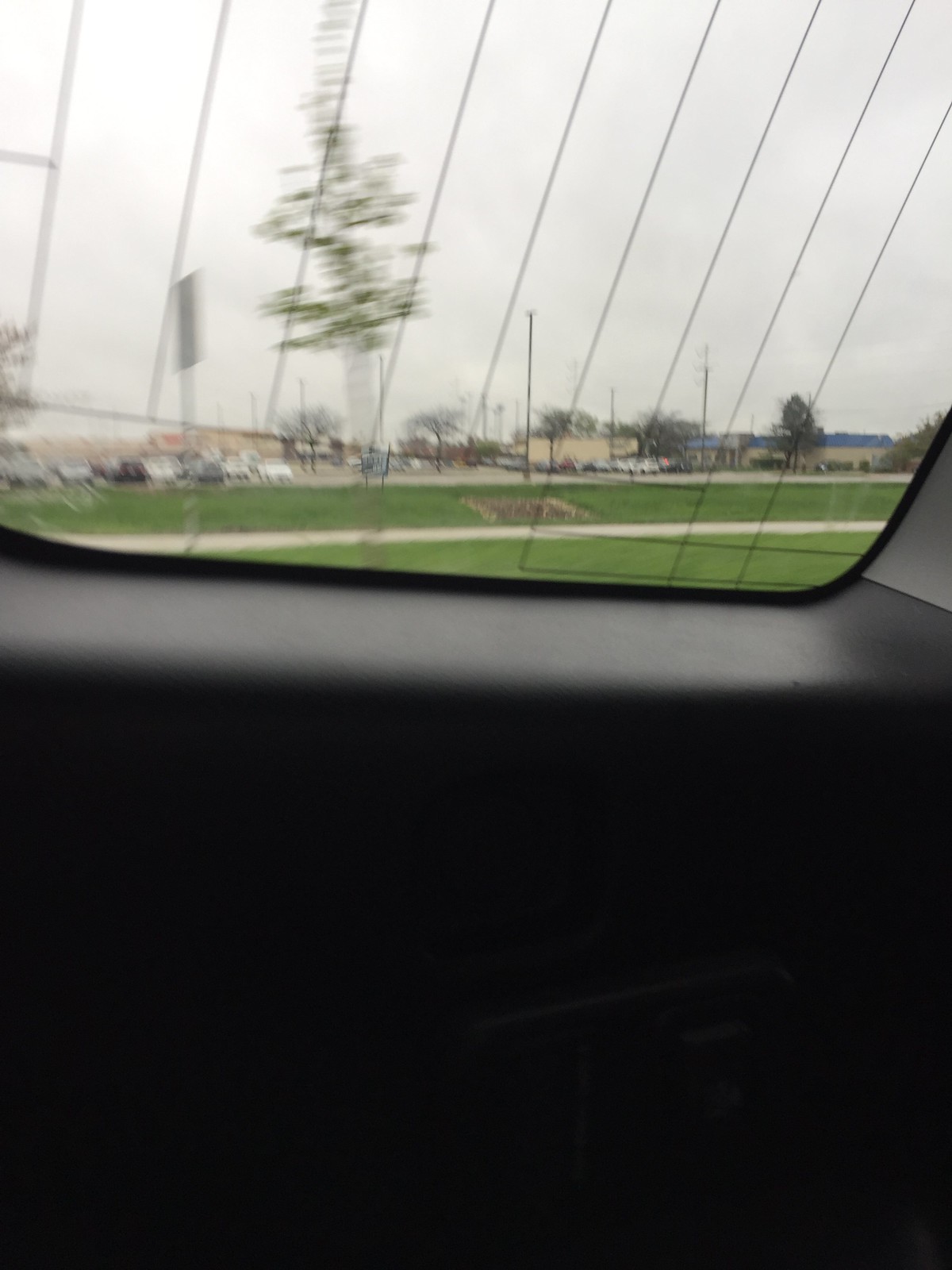An out-of-focus photograph taken from inside a car captures the view through a rear window adorned with a vertical defrosting grid pattern, subtly tilted to the right. The base of the window, shiny and curving slightly, is visible at the bottom of the image. Outside, a grassy area stretches beyond the window, leading to an industrial or retail setting. Out-of-focus cars are discernible on the left, while tan-colored buildings populate the right side of the background. The sky above is overcast, indicated by the gray clouds. In the center-left portion of the scene, a large object with green foliage, possibly a tree, adds an element of nature to the otherwise urban environment.